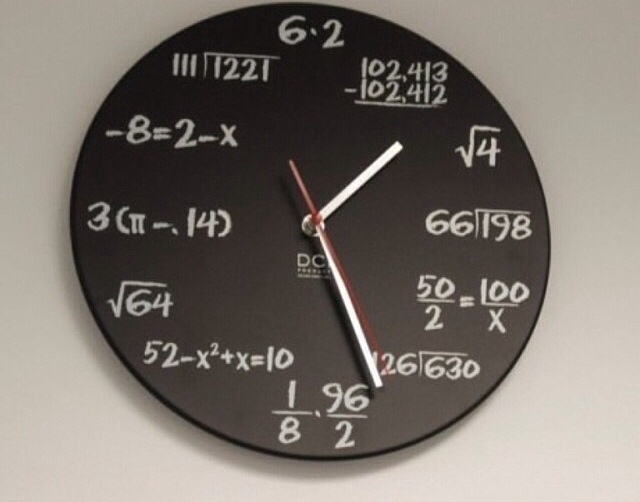This is a color photograph of an unusual analog clock mounted on a gray wall. The clock features a black background with large white numbers replaced by various mathematical equations written in white, which must be solved to determine the corresponding hour. Among the equations, at the very top where 12 should be, we see "6 × 2". Moving clockwise, at the position of 1 o’clock, it's "102,413 - 102,412" and at 2 o’clock, "198 ÷ 66". The clock continues with "50 ÷ 2 = 100 ÷ x" at 4 o’clock and "1/8 • 96 ÷ 2" at the bottom where 6 o’clock should be. The left side of the clock includes "-8 = 2 - x" at the 7 o’clock position and "3 lines beside each other divided into 1,221" at 9 o’clock. The hands of the clock are also noteworthy: the minute and hour hands are white while the second hand is light pink. At the center of the clock, there's the text "DC" and another indistinguishable word. The overall effect is a fusion of timekeeping and algebra, making it both a functional clock and a mathematical puzzle.